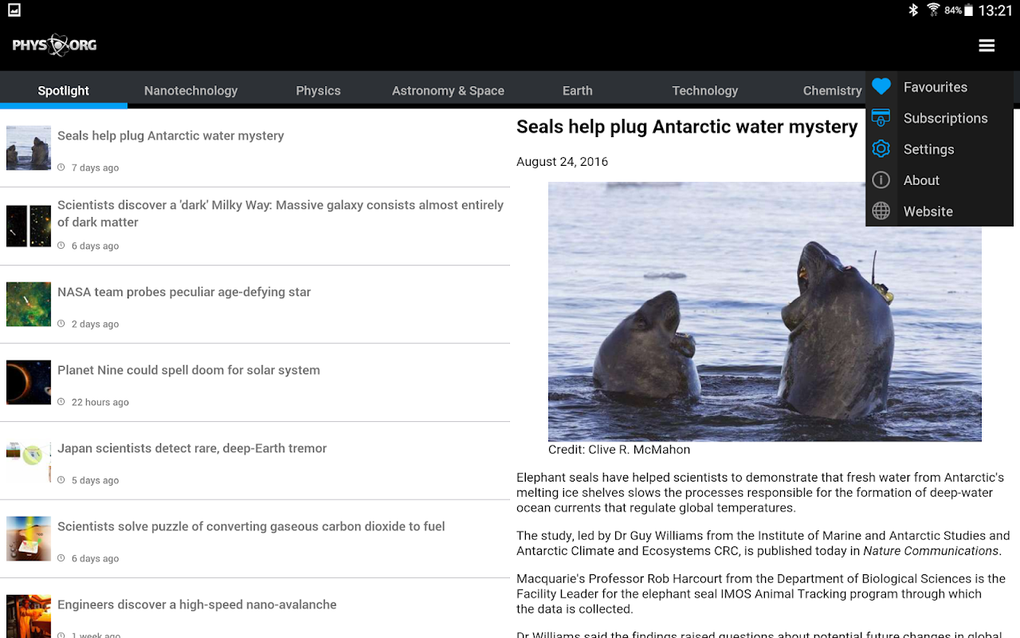The webpage displayed features the Phys.org logo at the top, followed by a navigation bar with tabs labeled Spotlight, Nanotechnology, Physics, Astronomy and Space, Earth, Technology, and Chemistry. To the right, there are icons for Favorites (a blue heart), Subscription (a subscription icon), Settings (an about icon), and Website (a website icon).

Central to the page is a vibrant image of two seals with their heads poking out of the water, each with their mouths wide open. The accompanying article is titled, "Seals Help Plug an Arctic Water Mystery." The content of the article highlights a breakthrough where elephant seals have aided scientists in revealing that the influx of fresh water from melting Antarctic ice shelves is decelerating the formation of deep-water ocean currents, which play a crucial role in regulating global temperatures.